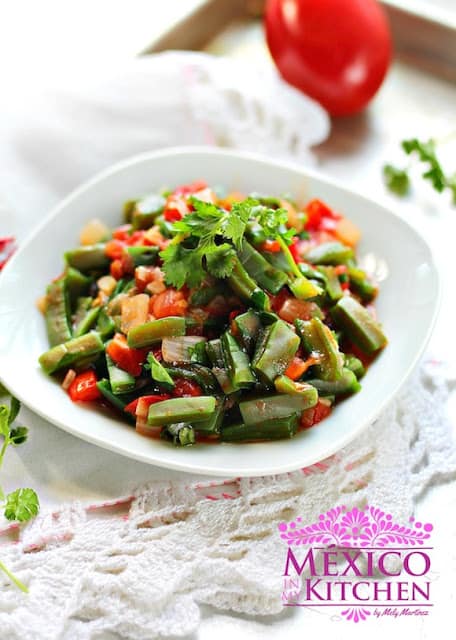This photorealistic image features a vibrant bowl of pico de gallo, showcasing a colorful mix of diced tomatoes and sliced peppers, topped off with a sprinkle of parsley. The food is artfully presented in a small, white ceramic bowl that sits atop a delicate crochet fabric, adding a homey touch. The setup rests on a large silver sheet pan, creating a stark contrast with the intricate fabric beneath. In the blurred background, a fresh tomato and some leafy cilantro add to the authentic feel of the scene, emphasizing the fresh ingredients used. Both bottom corners of the image display a light pink floral logo, each accompanied by purple text reading "Mexico Kitchen by Molly Martinez."